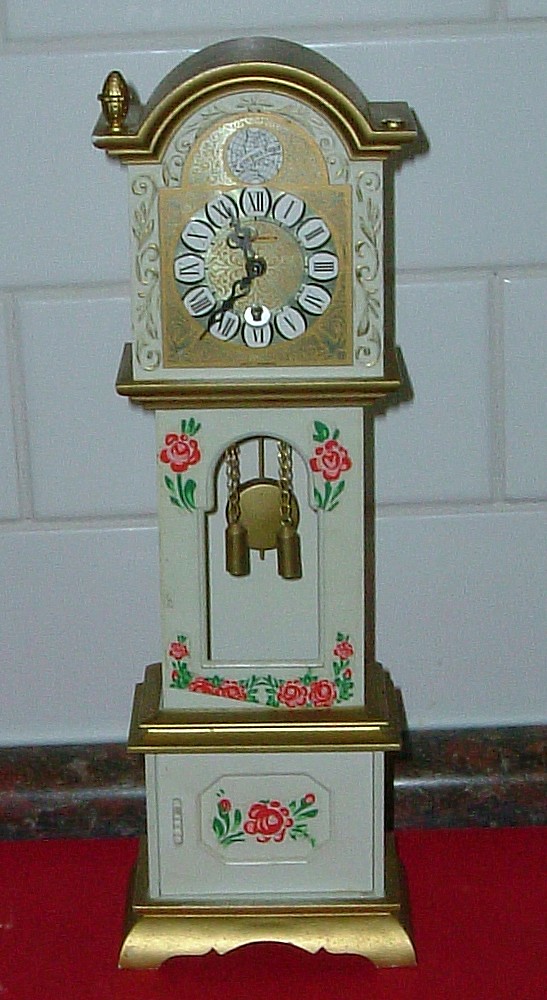This indoor photograph captures a charming vignette featuring a miniature grandfather clock against a white brick wall. The base surface resembles a plush red carpet, creating a warm and elegant backdrop. The clock’s casing is predominantly white, adorned with delicate red flowers and verdant green leaves. Its top section is decorated with intricate gold floral patterns. The clock face is a striking gold with small white circles housing black Roman numerals, and ornate minute and hour hands. Gold pendulums are visible through a glass pane in the middle of the clock. Crowning the piece is a regal gold egg ornament, adding a touch of opulence to this finely detailed miniature timepiece.